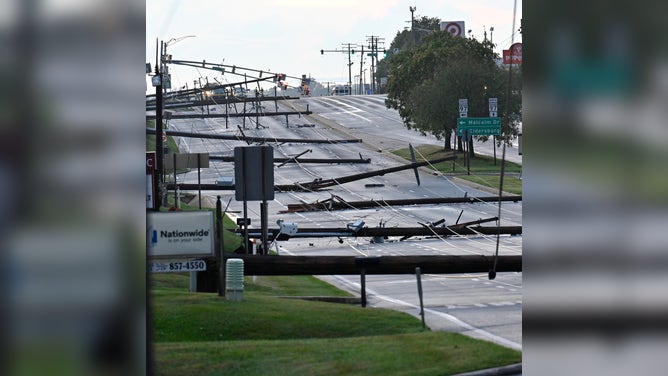A street, captured from a distance and seemingly taken with a cell phone, appears to be relatively free of cars but is marked by the aftermath of a natural disaster, potentially a hurricane or tornado. The road, grey in color and wet as if it has recently rained, is littered with fallen power poles and downed electrical wires, creating a domino effect along the left side. These poles, some of which look as if they are waiting to be replaced, have tangled the street in a hazardous mess. Large patches of green grass are visible on both sides, with a circular median on the right topped by a set of trees. In the backdrop, several signs are discernible, including a blue "Nationwide" sign with the phone number "857-4550," a Target store sign, and a red Popeyes sign. A green interstate sign displaying confusing speed limits (97, 67, or 47 miles an hour) is also present but hard to read. Among the chaos, a street sign indicates "Malcolm Drive," adding to the scattered details of the scene. Overall, the photo shows extensive damage and debris, indicating a significant cleanup ahead amidst an otherwise serene, verdant neighborhood.